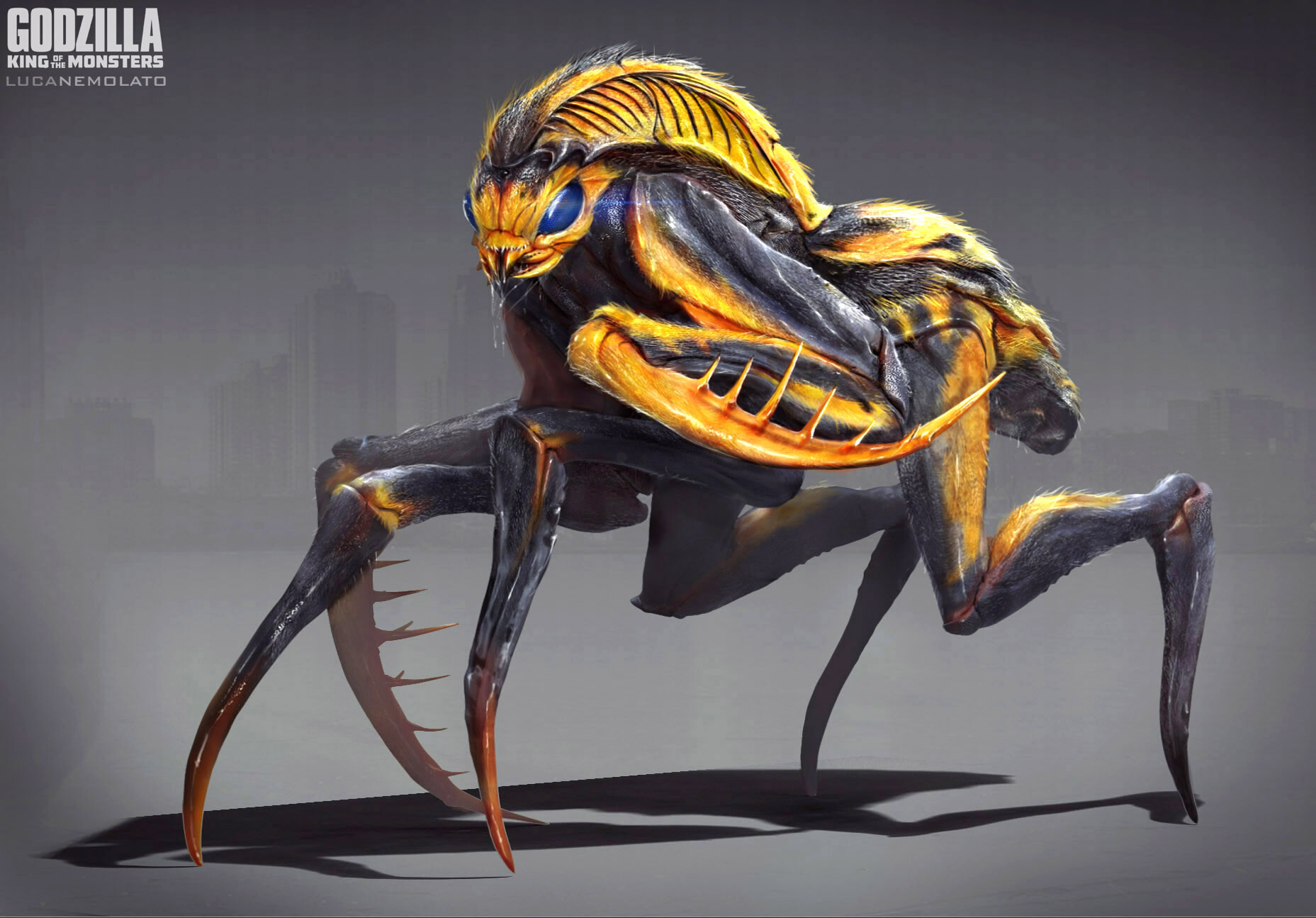This image features detailed concept art of a monster from "Godzilla: King of the Monsters." Displayed in the top left corner are the film's title and the name "Luca Nemolata," possibly the artist. The creature stands out with its menacing, insect-like appearance, combining elements of various arthropods. It features a black and yellow color scheme accentuated with red bits. The body resembles that of a bee, the face mirrors a wasp with pronounced yellow and black markings, and it has large, intimidating eyes. The creature has four spider-like legs and two mantis-like arms armed with sharp, knife-like spikes. Drool drips from its predator-style mouth, further enhancing its fearsome look. The monster's overall posture and elements evoke a sense of an otherworldly insect amalgamation, exuding both menace and fantasy.